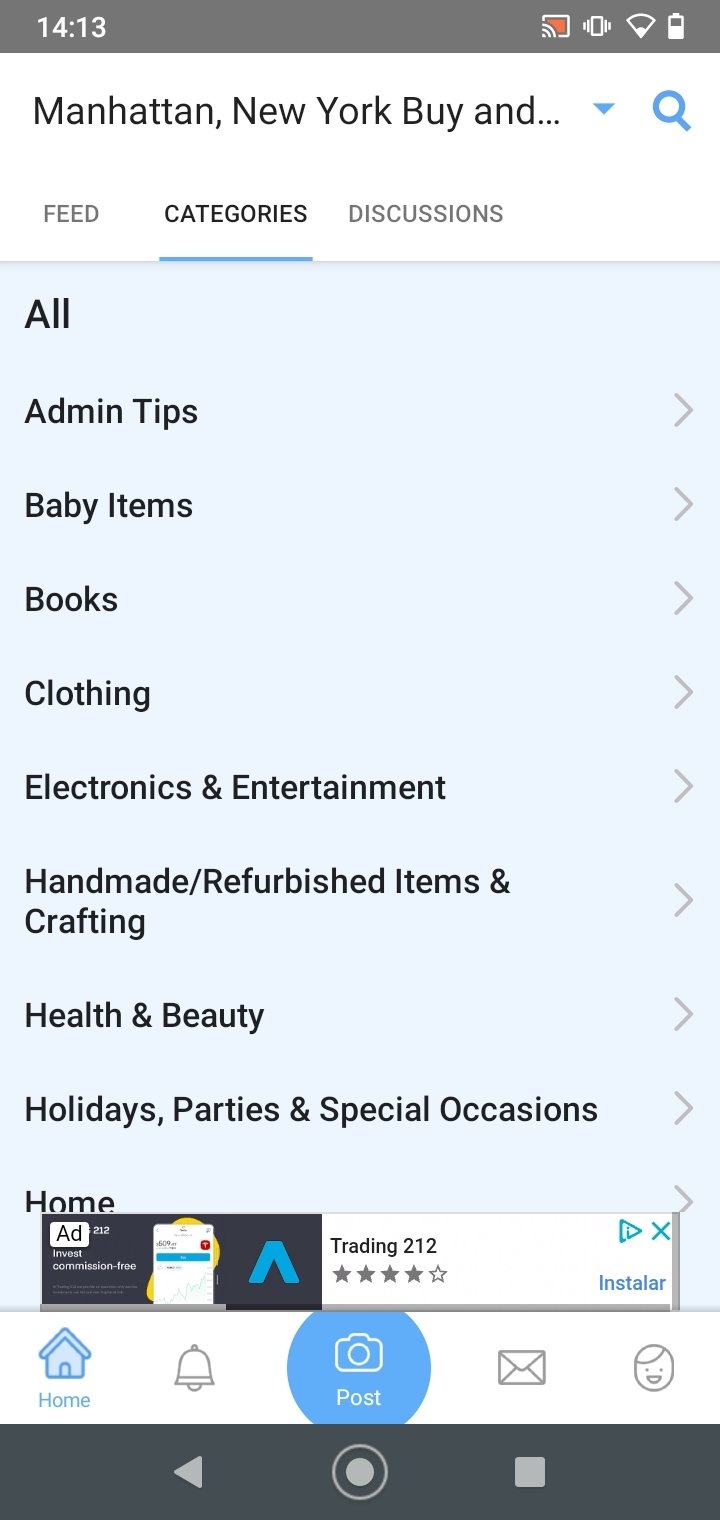This image depicts a tablet screen displaying its interface at 14:13 military time. The battery life indicator shows as full, denoted by being in the white. However, the Wi-Fi connection appears to be weak. Below the status bar, the location reads "Manhattan, New York" with a small dot and is accompanied by a blue drop-down arrow and a blue magnifying glass icon for search functionality.

Directly underneath this, there are three tabs labeled 'Feed', 'Categories', and 'Discussions', with the 'Categories' tab selected and underlined in blue. The 'Categories' section presents a list of options, each followed by a rightward arrow for further navigation. The options are as follows: 'All', 'Admin Tips', 'Baby Items', 'Books', 'Clothing', 'Electronics and Entertainment', 'Handmade, Refurbished Items and Crafting', 'Health and Beauty', 'Holidays, Parties, and Special Occasions', and 'Home'.

An advertisement banner appears at the bottom of the screen, interrupting the categories. This detailed snapshot provides a clear view of the tablet's interface and its organizational features at the specific moment captured.